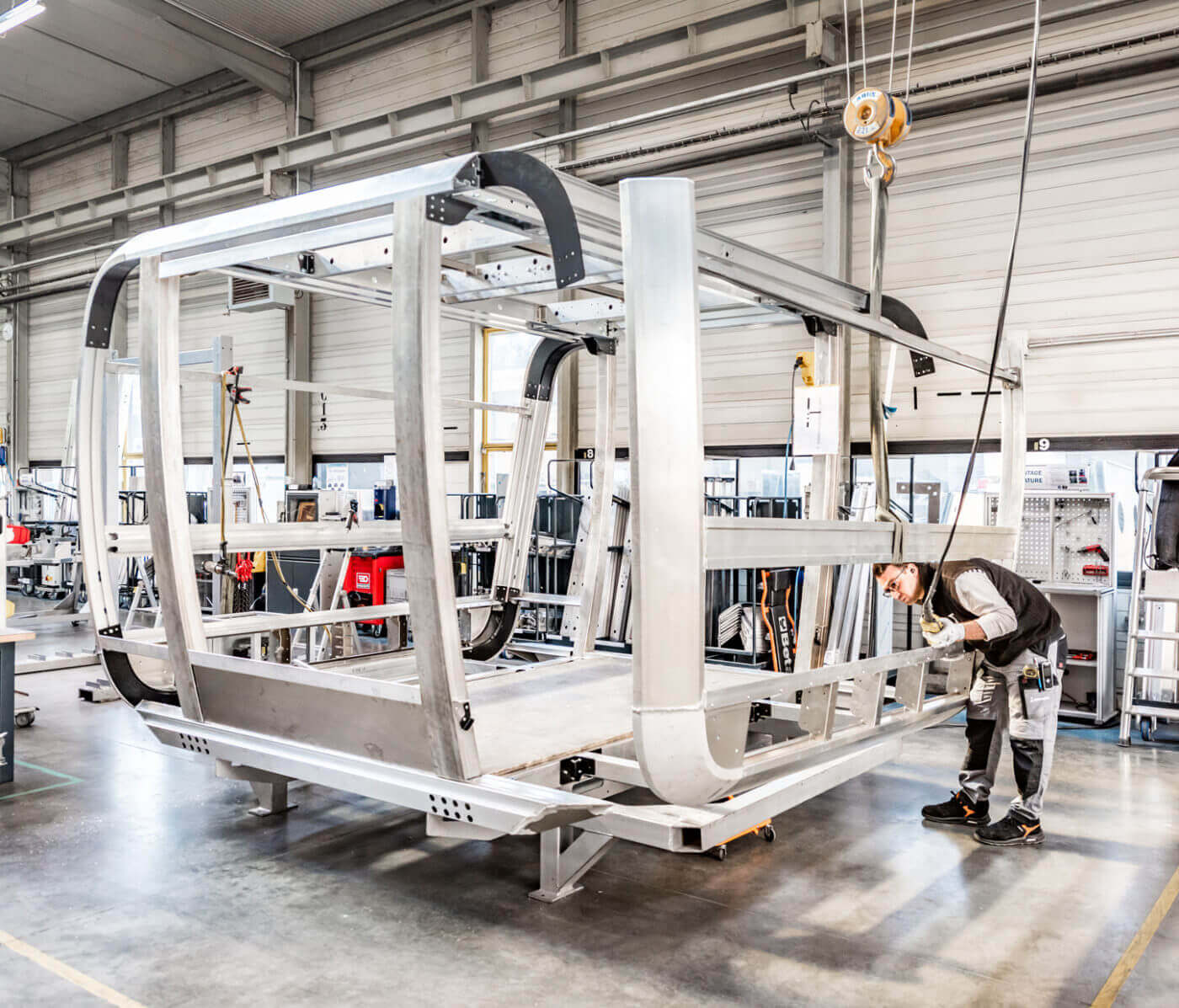In a spacious, industrial garage with high ceilings and partially open metal doors, a man is intently working on a large metallic framed device that resembles the skeleton of a trailer. The concrete floor beneath him is marked with prominent yellow border stripes. The man, wearing a black vest over a white shirt, white pants with black accents, and black shoes, is bent over the device with one gloved hand visible. He is carefully manipulating wires that descend from the ceiling towards the metallic structure. This setting, filled with the machinery and equipment indicative of a factory, features a puller and levy system aiding him in his task. The detailed scene highlights the technical environment and the focused effort of the individual as he inspects and interacts with the mechanical apparatus.